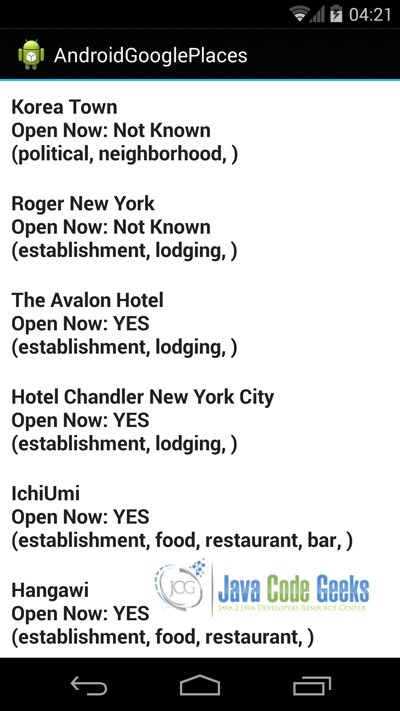Here is a restructured and detailed caption for the image:

"A screenshot of a smartphone displaying various information. The status bar at the top shows Wi-Fi and cellular bars, the charging icon, and the current time, 4:21. This is presented on a black banner. Below the status bar is the Android Google search bar, featuring a small Android icon.

The main content area, on a white background with black text, lists several establishments in New York City:

1. **Koreatown:**
   - Status: Open Now
   - Category: Not a political neighborhood
   - Details: Comment in parentheses indicates it's specifically "Roger New York."

2. **The Avalon Hotel:**
   - Status: Open Now
   - Category: Lodging Establishment

3. **Hotel Chandler:**
   - Status: Open Now
   - Category: Lodging Establishment

4. **ICH UMI:**
   - Status: Open Now
   - Category: Food, Restaurant, Bar

5. **Hangawi:**
   - Status: Open Now
   - Category: Food, Restaurant

Next to "Hangawi," there is a mention of "Java Code Geeks" in blue and green text, which changes color to white.

At the bottom of the screen is a black navigation bar featuring a left arrow, a home icon, and a copy icon."